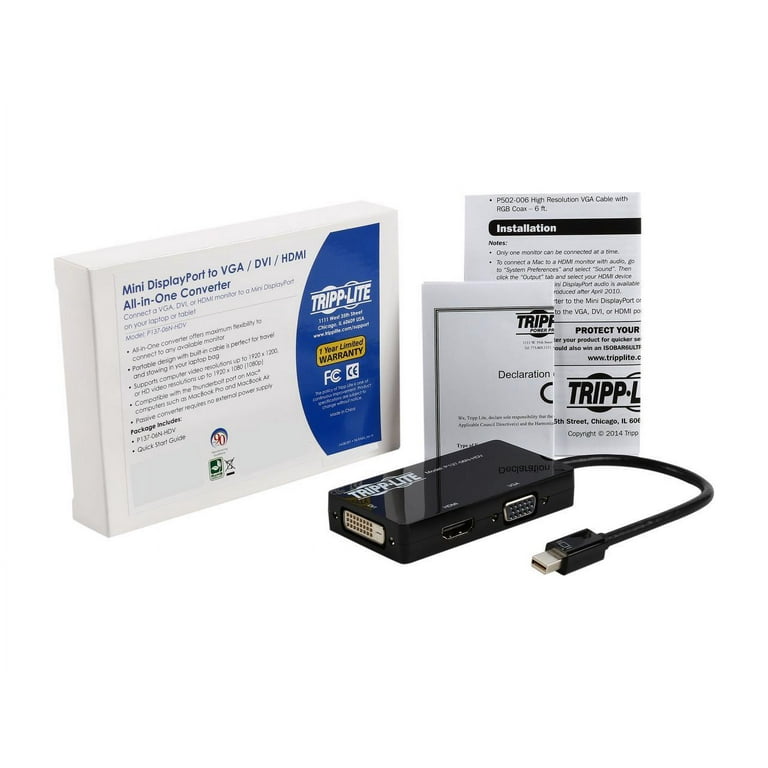This is a professional photograph of an electronic device, specifically a computer accessory that serves as a Mini DisplayPort to VGA, DVI, and HDMI all-in-one converter. The central focus of the image is a shiny, rectangular black box labeled "Tripp Lite." This device has a short USB cable extending from its back. The box contains an HDMI plug and VGA plus DVI adapters on its sides. Behind the device lies its packaging, which is predominantly black, white, blue, and yellow. The packaging clearly states the product's purpose and features, including "Mini DisplayPort to VGA/DVI/HDMI All-in-One Converter" and a "One Year Limited Warranty." To the right side of the device, you can also see the folded instruction manuals, which include installation details and a declaration from Tripp Lite. Although some smaller text is present, it is too small to be read clearly.